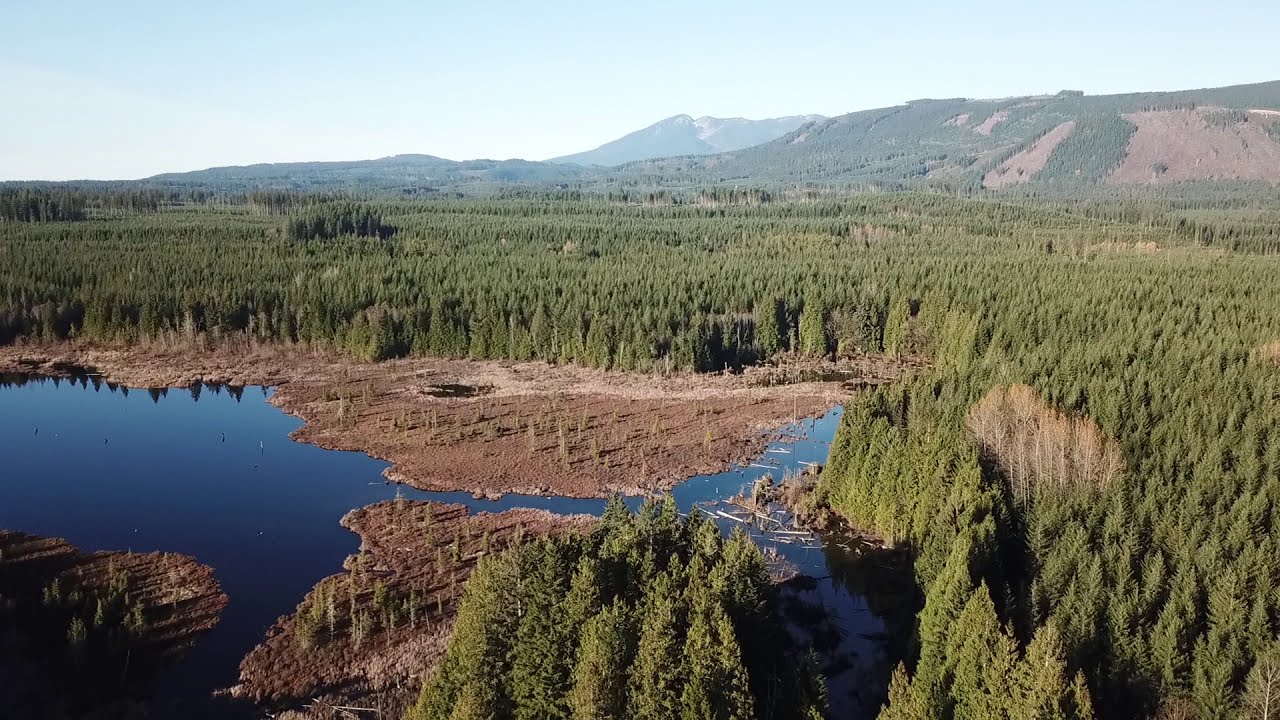This aerial photograph captures a stunning coniferous forest landscape with occasional deciduous trees interspersed. In the lower left-hand corner, a small lake or pond, bordered by brown muddy shores and saplings, makes its way into the edge of the forest. Logs and branches float in the dark, gradient blue water, adding a rustic charm to the scene. The forest stretches out over undulating land, leading up to low mountains or hills in the background, likely around 300 feet tall. These elevations are sparsely covered with trees, showing signs of clear-cutting or natural rocky patches where vegetation struggles to grow. Some areas within the forest display bare ground, possibly from reforestation efforts or water-induced tree dieback. The picturesque setting is completed by a light blue sky with thin, wispy clouds overhead. This tranquil scene represents a lush wetland area, possibly located in the far north or northwest, devoid of visible human or animal presence from this height.